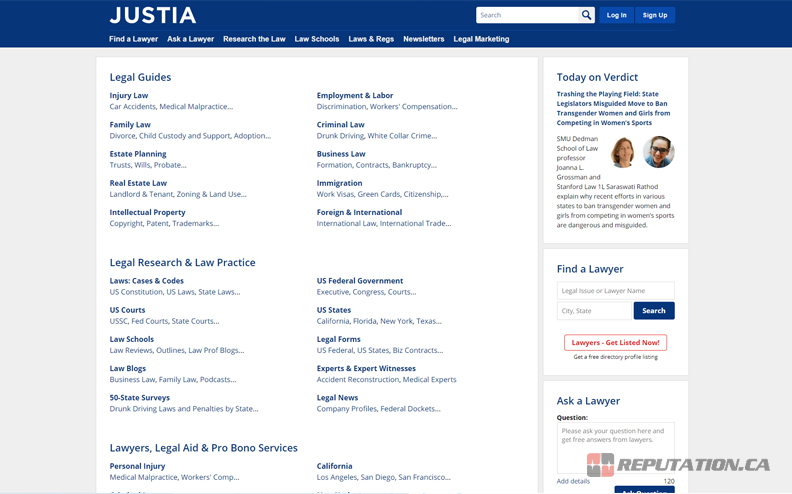The image captures the homepage of the Justia website. At the top-left corner, slightly indented from the left edge, the Justia logo is prominently displayed within a horizontal blue menu bar that spans the width of the page. This blue bar also functions as a navigation menu, with a search bar located at the top-right corner, flanked by a "Login" button to its immediate right, and a "Sign Up" button further to the right of the "Login" button. 

Directly beneath the Justia logo, the horizontal menu offers several navigation options in white font: "Find a Lawyer," "Ask a Lawyer," "Research the Law," "Law Schools," "Laws and Regs," "Newsletters," and "Legal Marketing."

The primary section of the website, set against a white background, features a sidebar on the left with various links. The sidebar includes categories such as "Legal Guide," "Legal Research and Law Practice," as well as "Lawyers," "Legal Aids," and "Pro Bono Services."